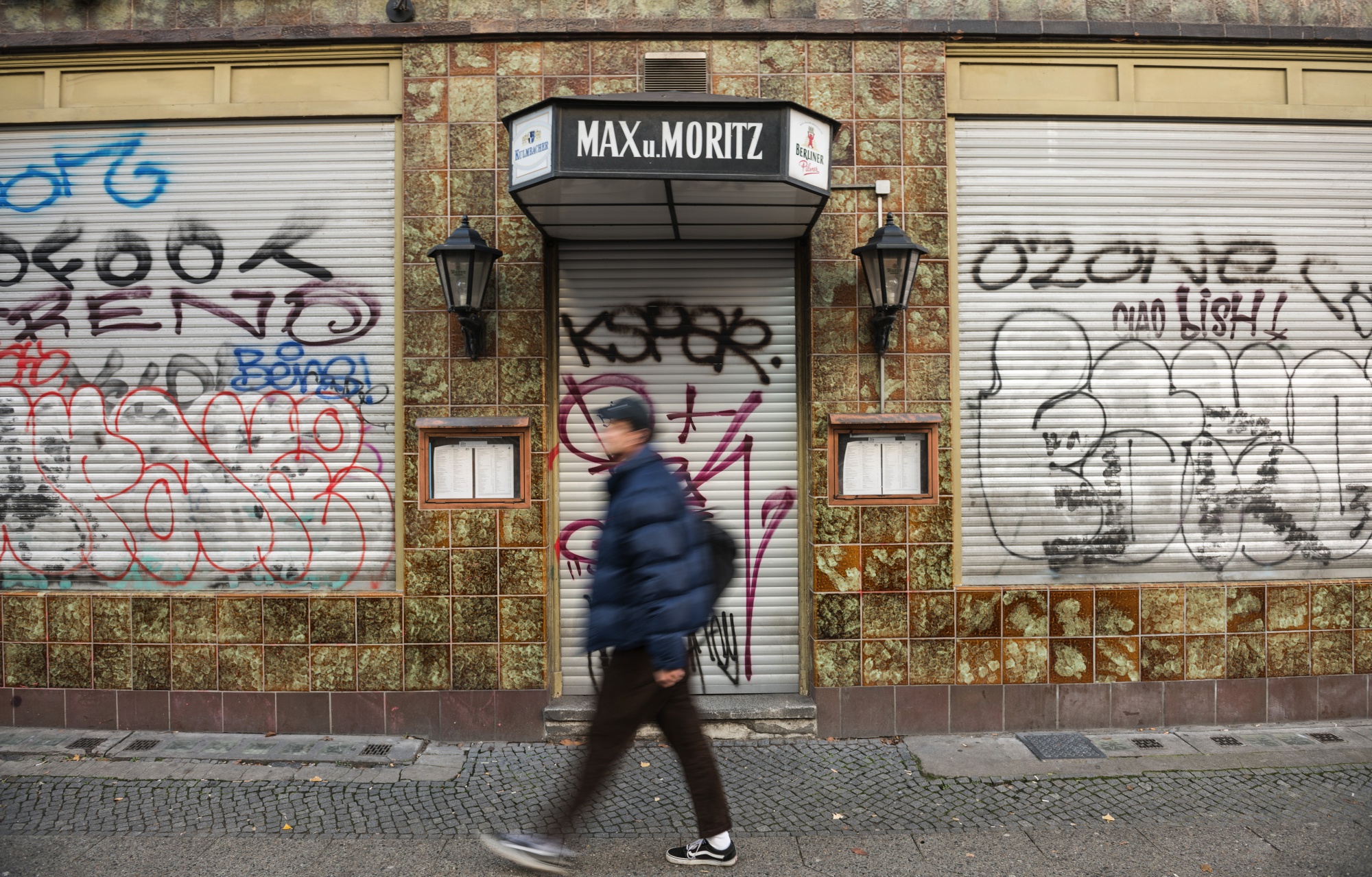In this vividly detailed photo, a man in a blue puffy jacket, black sneakers, and black pants is caught in motion, creating a slight blur as he walks briskly down a desolate street. His face is not clearly visible, but he appears to be of Asian descent. The setting features a closed-down building with a centered door marked by a sign above it that reads "Max U. Moritz," indicating it might be in a foreign country. The building has two large windows with blinds and metal gates, one on either side of the door. These gates, along with the door, are heavily adorned with various colorful graffiti in shades of black, purple, blue, and red. The wall surrounding the door is covered in tiles with a blotchy rust and greenish hue, contributing to the overall decrepit appearance of the scene. Lamps flank the sign, and the names "chalvish" and "ozone" can be discerned amidst the myriad of graffiti tags, adding to the feeling of urban decay.